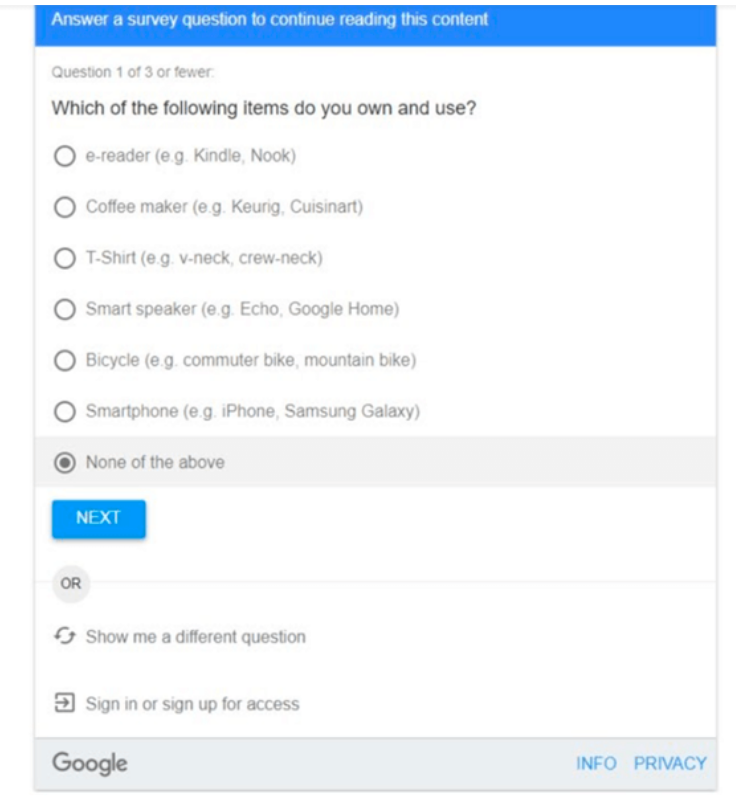The image depicts a Google pop-up advertisement that appears when attempting to access certain articles. The pop-up features prominent blue borders and white text that reads, "Answer a survey question to continue reading this content." At the top, it indicates "Question 1 of 3 or fewer" in a slightly gray text. Below this, in larger, bold black text, it asks, "Which of the following items do you own and use?" 

Presented underneath in a vertical list are multiple-choice options including "e-reader (e.g., Kindle)," "Coffee maker (for Keurig or Cuisinart)," "T-shirt," "Smart speaker," "Bicycle," or "Smartphone." There's also an option labeled "None of the above," which, in this instance, has been selected. Upon selecting an option, the chosen button turns black, while the "Next" button below it is displayed in blue.

Further down, a gray circular button with a refresh icon offers an option to "show me a different question". To the left, a small text indicates options to "Sign in or Sign up for access."

At the very bottom, a gray bar spans the width of the pop-up, displaying "Google" in black on the bottom left, and "INFO" and "PRIVACY" in blue, all capitalized, on the far right. This survey is part of Google’s strategy to collect user preferences to tailor advertisements more effectively.